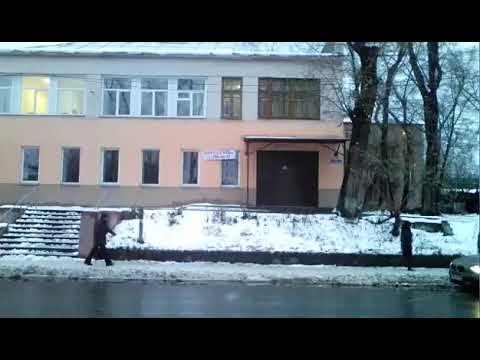In this image, a person dressed in black is walking down a snow-covered pavement toward a car with its headlights on. The scene is set in front of a two-colored house, with a pink bottom part and a white top part. The house, which may be on a slight hill, features several steps leading up to the entrance. The roof, walls, and steps are blanketed in snow, contributing to the overall wintry atmosphere. Despite the snow, one room in the house is lit, casting a warm glow through the windows, while the entrance appears dark and possibly closed. Surrounding the house are several leafless, dry trees. The wet road and the snow-laden environment accentuate the chilly weather.